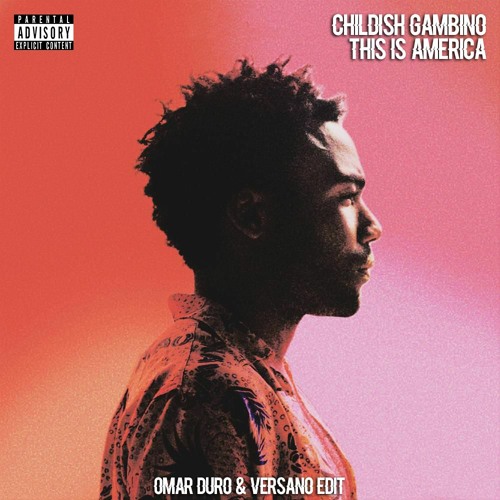The image depicts an album cover with a distinctive pink-to-deep red gradient background, starting light on the right and turning darker towards the left. Dominating the center is a side profile of Childish Gambino, also known as Donald Glover, who gazes seriously to the right. He is dressed in a red and black Hawaiian-style shirt, and his short, slightly spiky hair frames his intense expression. In the top right corner, white text reads "A Childish Gambino - This is America," while the top left corner features the traditional black and white "Parental Advisory Explicit Content" sticker. At the bottom of the image, more white text credits Omar Duro and Versano Edit. The overall design is minimalistic, with no additional figures or elements, focusing entirely on Gambino and the pertinent textual details.